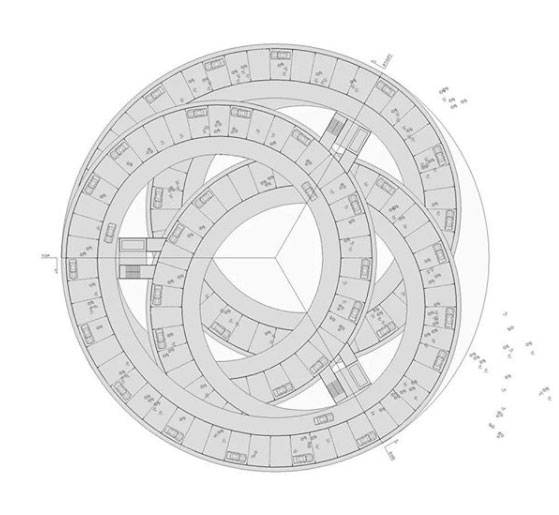The image depicts a detailed, intricately coiled, black-and-gray circular diagram, reminiscent of a measuring tape or curved ruler, centrally placed on a pristine white background. This diagram, characterized by its lack of a definable border, features numerous segments adorned with a mixture of blocks, numbers, and symbols. It spirals inward, forming concentric circles, akin to a snake coiled upon itself. Scattered around the central coil are additional markings and possible formulas, though they appear indecipherable. Three faint, pencil-like lines radiate from the center, creating a star-like pattern overlaying the diagram. The overall composition suggests a scientific or educational setting, embodying an abstract, methodical design that hints at complex, possibly mathematical, purposes.